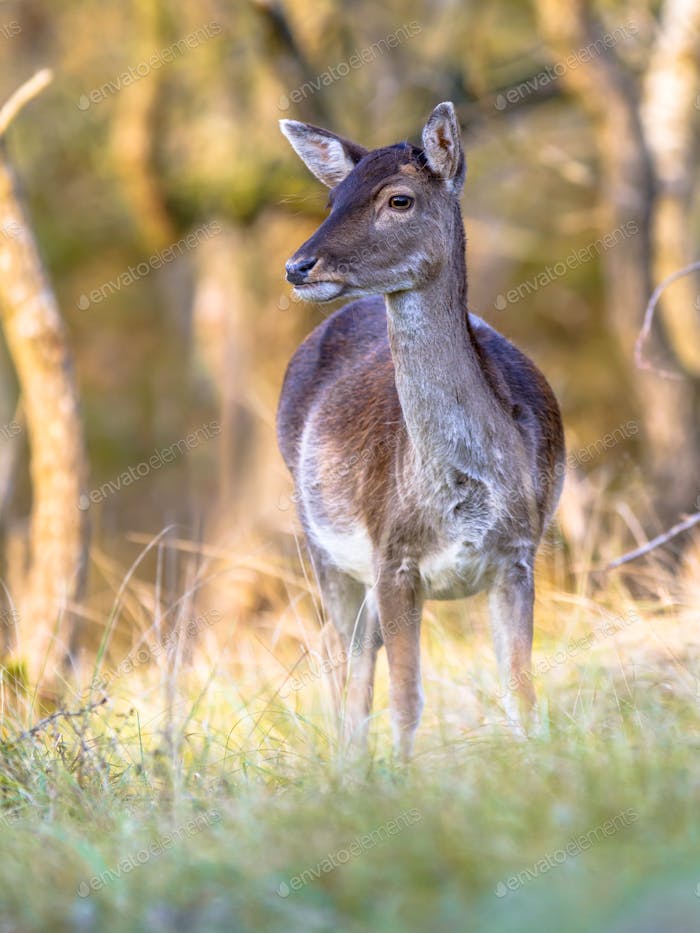The image captures a small, bewildered deer with a brown coating on its fur and a long neck, standing amidst disheveled green grass in a forest-like area. The deer, which lacks horns and has only its left eye visible to the camera, faces slightly left, allowing a clear view of its black nose and black pupil. The background features several thin, leafless tree trunks, each approximately 8 to 10 inches in diameter. A watermark from Envato Elements runs faintly across the image, adding a subtle grid of copyright text over the photograph. All objects in the image maintain an upright angle, and the focus is primarily on the deer, with the surrounding elements slightly blurred to emphasize the animal's presence.